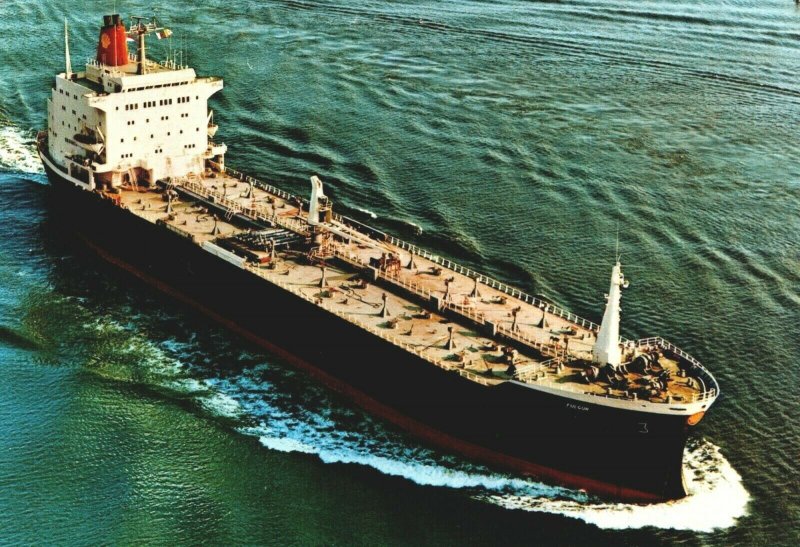This is a high-resolution, color landscape photograph captured from a drone, providing an aerial view looking down at a large merchant Navy tanker ship cutting through dark green waters tinged with bluish and yellow hues. The ship is oriented diagonally, with the bow facing the bottom right corner and the stern angled towards the top left. The ship features a prominent multi-story cabin structure at the stern, which is white with five levels, topped by a large, red exhaust plume emitting black fumes and an antenna pole in front. The deck is beige with various metallic poles and structures, including two white towers; one is situated near the bow, likely a radar or communication pole, and the other is towards the middle of the ship. The ship’s side is black with a red line along the bottom, and the number '3' is clearly visible in white near the bow, surrounded by other smaller, unreadable text. The foamy wake created by the bow as it cuts through the water adds to the dynamic realism of the scene, highlighting the intricate details and the scale of the vessel against the vast ocean.